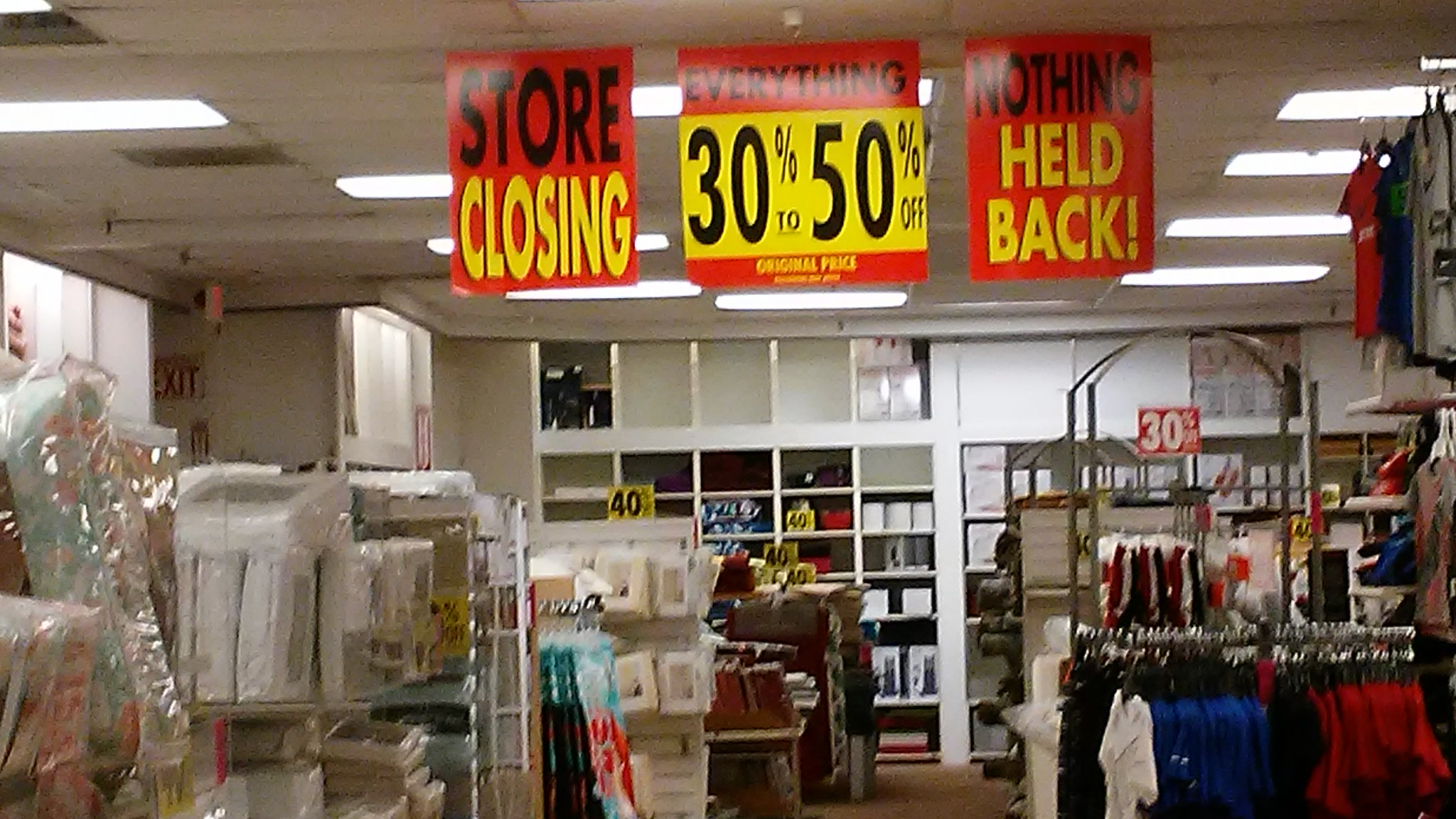This image captures the interior of a store that is in the process of closing down. The ceiling features acoustic tiles with recessed lighting that appears to consist of outdated fluorescent fixtures. Three prominent signs hang from the ceiling. The first sign has a red background with "STORE" written in bold black capital letters at the top, and "CLOSING" displayed in bold yellow capital letters at the bottom. The second sign also has a red background, with "EVERYTHING" in bold black capital letters at the top, "30 TO 50% OFF" in the middle on a yellow background with a red and black font, and "ORIGINAL PRICE" in bold yellow capital letters at the bottom. The third sign follows a similar design, featuring "NOTHING" in bold black capital letters at the top, "HELD" in yellow capital letters in the middle, and "BACK!" in bold yellow capital letters at the bottom.

To the left of the image, there are shelves stocked with bedding or baby items in white, pink, and blue colors. On the right-hand side, a rack displays smaller T-shirts in white, blue, and red. Behind this rack is a shelf that appears to hold hanging underwear. Further to the right, higher shelves display more small T-shirts in white, navy, and gray, some of which feature printed designs.

In the far background, a series of labeled cubbies indicate a 40% off discount with yellow signs. These cubbies seem to contain jars, which might be for spices, grinders, or possibly baby food makers. The overall scene conveys a sense of clearance and finality as the store prepares for its closure.